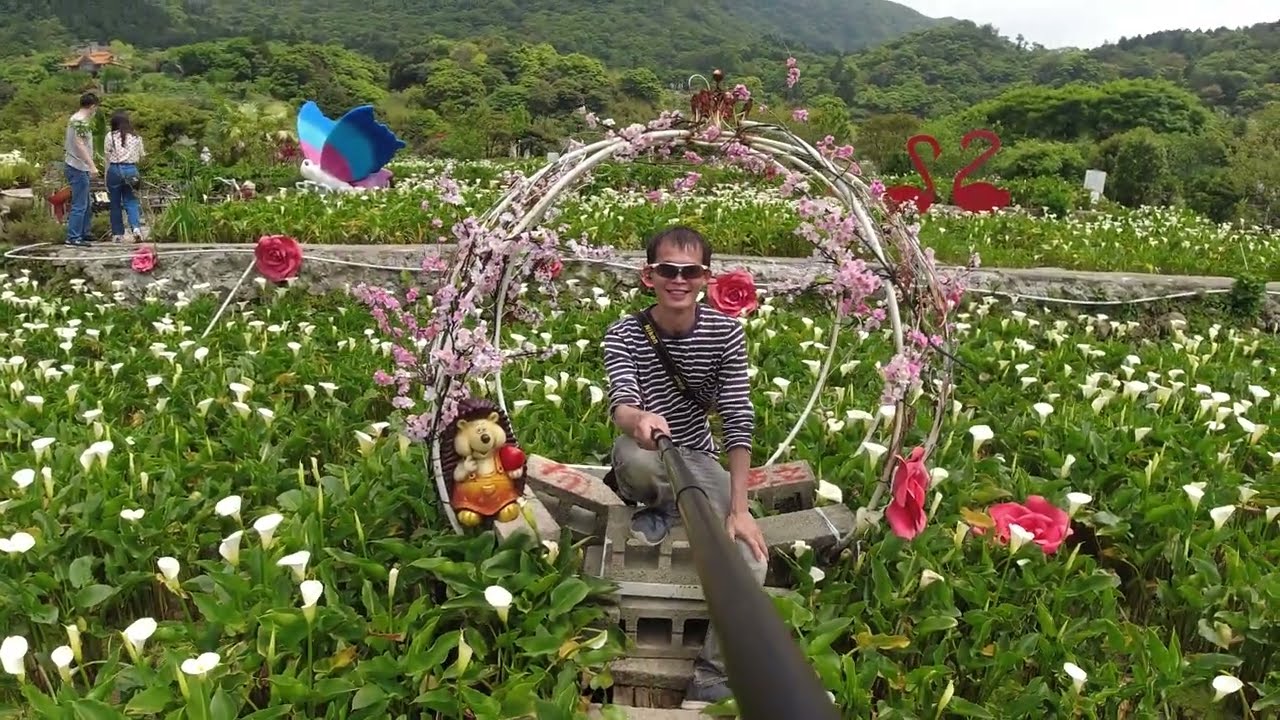The photograph captures a cheerful young man of Asian descent taking a selfie in an outdoor garden using a selfie stick, clearly visible in the image. He has short, thinning black hair and brown skin, and he is wearing sunglasses along with a black and white horizontal striped long-sleeve shirt, gray pants, and gray sneakers. A yellow and blue crossbody strap suggests he may be carrying a bag. The man is seated on a circular structure made of cinder blocks, surrounded by lush greenery and white calla lilies with green stems. Encircling him, there are two sets of hoops adorned with pink flowers, and a stuffed hedgehog toy is placed on the lower left side of the hoop. On his right, there are two pink flamingo statues, and to the left, a whimsical display featuring metal flowers and a blue and pink winged white butterfly. Further into the distance, towards the left, a man and a woman dressed in white or gray shirts and blue jeans are visible, standing on a stone walkway. Behind them, the dense forest stretches into tree-covered hills, completing the serene and picturesque scene.